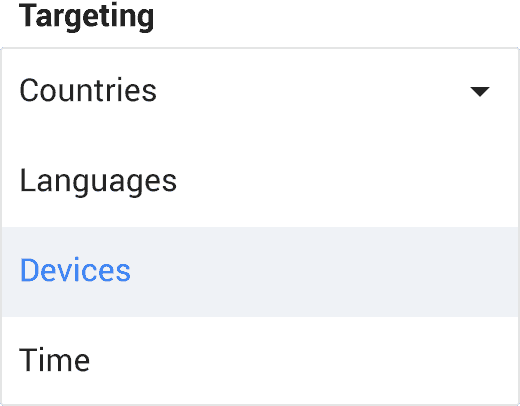This screenshot exhibits a minimalist design with a predominantly white background and just five lines of text, making its user interface simple and intuitive. At the top, the bold, black text reads "Targeting." Below it, there is a rectangle outlined with a thin, light gray line. Inside this rectangle, the first line of black text reads "Countries," accompanied by a downward-pointing triangle on the right-hand side, indicating a drop-down menu for more options.

Moving down, the left-aligned black text reads "Languages." The subsequent line, which stands out due to its blue lettering, reads "Devices." This "Devices" line is highlighted with a light gray background, emphasizing its selection. Finally, the last line of black text reads "Time." The overall layout and color scheme prioritize clarity and ease of use.